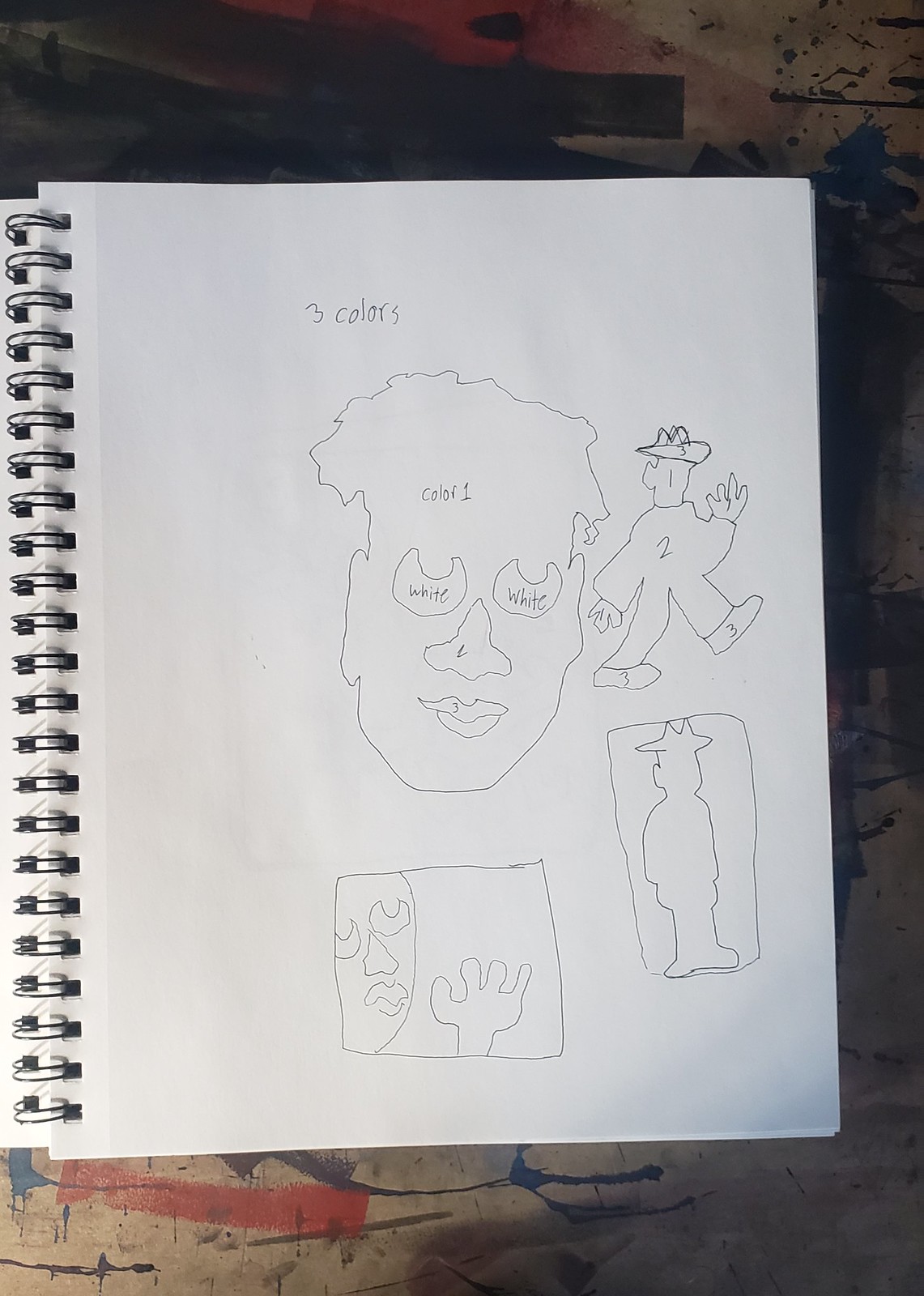In this image, we see a sketchbook opened to a specific page, revealing a meticulous drawing on its spiral-bound paper. The drawing appears to be created with thin lines, likely using pencil or pen, indicative of a preliminary sketch. The composition includes an outlined face labeled with "color 1" instead of being filled in, suggesting instructions for a coloring exercise. The eyes are marked with "white," and the nose and lips are numbered "2" and "3," respectively. Additionally, a figure resembling a body is sketched with numbers: "1" on the head, "2" on the body, and "3" on the feet. These annotations imply that the sketch is part of an art class assignment or instructional guide, providing detailed steps for coloring the drawing. The layout and labeling suggest an educational purpose, possibly to teach shading or color placement techniques.